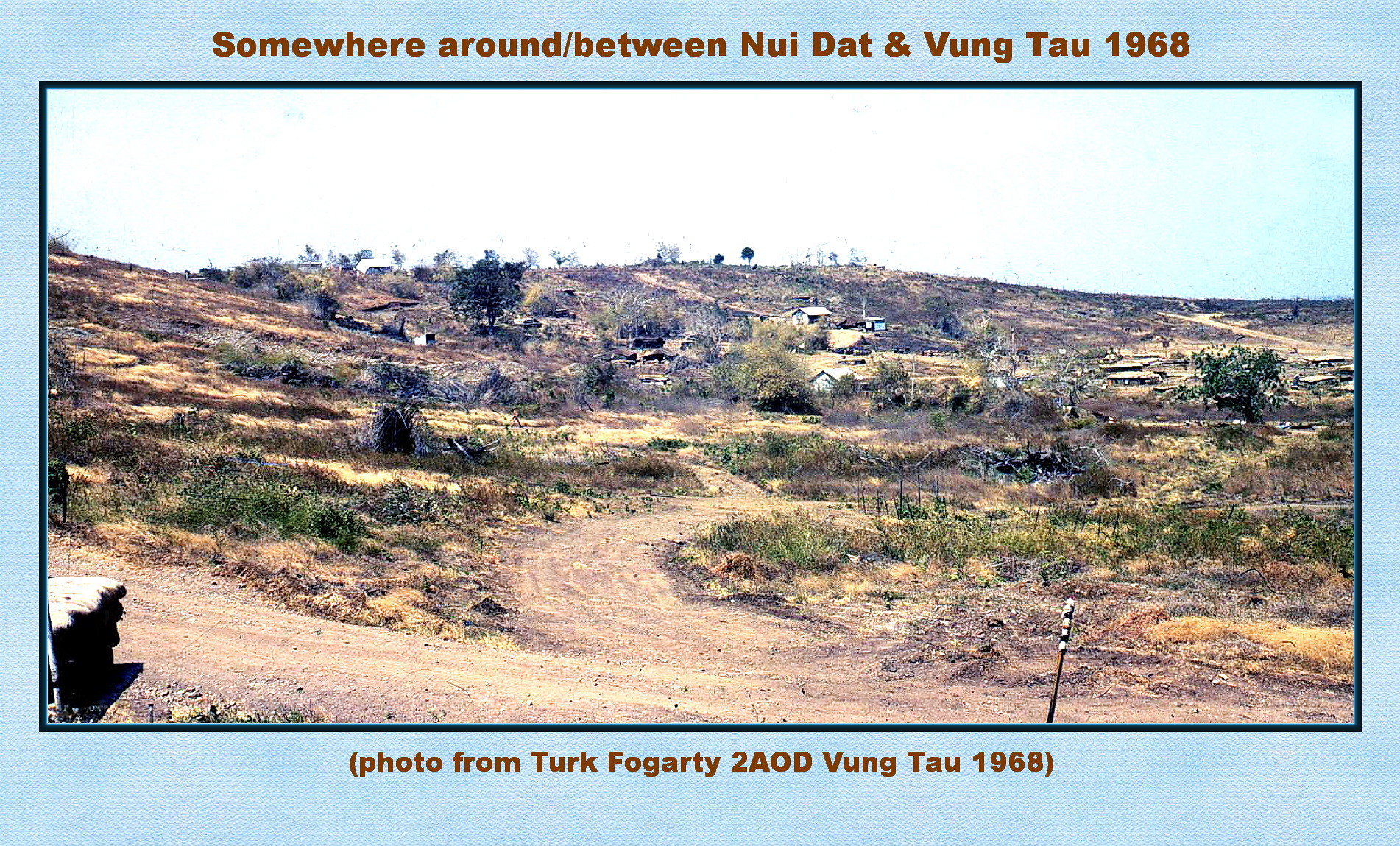This photograph, set against a light blue background with a black frame, captures a landscape likely in Vietnam circa 1968. It features red lettering above and below the image. The top caption reads, "Somewhere around/between Nui Dat and Vung Tau, 1968." The bottom caption states, "(photo from Turk Fogarty to AOD Vung Tau, 1968)." The image depicts a hillside with two dirt roads forking off from a main road in the foreground. Sparse vegetation including grass patches, shrubs, and small trees, some possibly burnt or dead, dot the landscape. Scattered across the hill are small, dilapidated houses or shacks, suggesting a village or encampment. The sky above is a bright blue, further enhancing the sense of place and time in this historical snapshot.